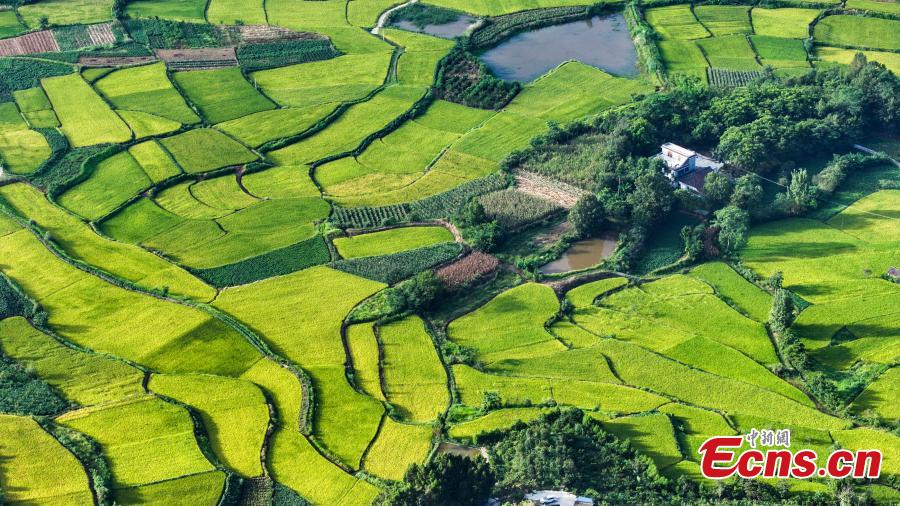This image presents a detailed aerial view of a sprawling, lush green field, showcasing an exquisite patchwork of varying shades of green—from vibrant light greens to deeper, olive hues. The photograph, likely captured by a drone, provides a bird's-eye perspective highlighting the intricate landscape and differing elevations of the terrain. Prominently on the right side of the image, a cluster of darker green trees encircles a lone, white house, creating an eye-catching focal point. Further enhancing the scene's idyllic charm, a small, serene pond sits near the top center of the frame. Additional areas reveal scattered crops suggesting a small farm. On the bottom right-hand corner of the image, the red text "ecns.cn" is visible, possibly indicating the source website. This well-lit daytime photograph captures a vivid snapshot of rural tranquility.